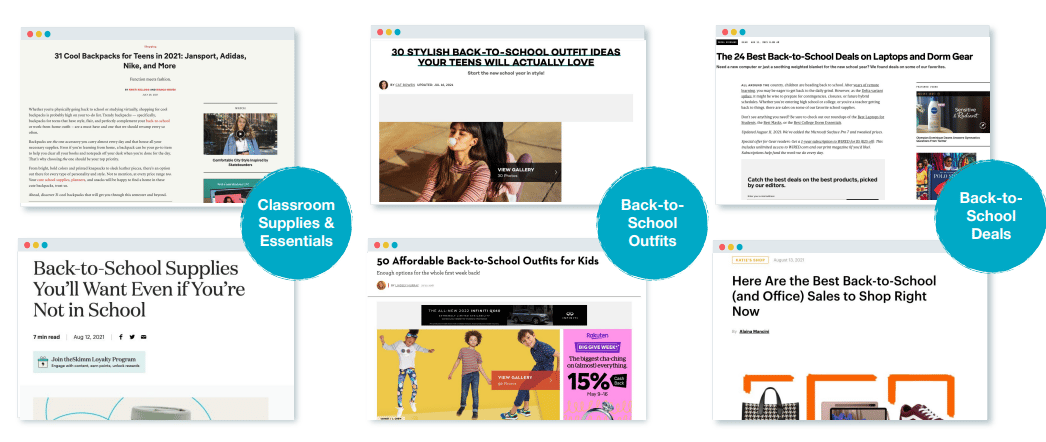This image is divided into several categorized sections, each denoted by a different colored box or circle. 

- **Top Section:** The uppermost square features the title "Cool Backpacks for Teens in 2021" followed by prominent brands such as Jansport, Adidas, and Nike.
- **Middle Section:** Below this, a text box highlights "Back to School Supplies You'll Want Even If You're Not in School." Positioned between these two sections is a blue circle titled "Classroom Supplies and Essentials."
- **Right Side:** Adjacent to the middle section, a similar title from the top appears emphasizing "30 Stylish Backpacks." Beneath it, another segment reads "50 Affordable Back to School Outfits for Kids" with a blue circle inscribed with the same, "Back to School Outfits."
- **Lower Right Section:** This area details "The 24 Best Back to School Deals on Laptops and Dorm Gear." Further down, it presents "The Best Back to School and Office Sales to Shop Right Now," accompanied by images of a purse, tennis shoe, and an iPad.
- **Final Blue Circle:** Near the bottom, the final blue circle elaborates on the category "Back to School Deals."

Overall, the image is a comprehensive, visually organized guide highlighting various back-to-school essentials and promotions for 2021, encompassing everything from trendy backpacks and outfits to electronics and accessories.